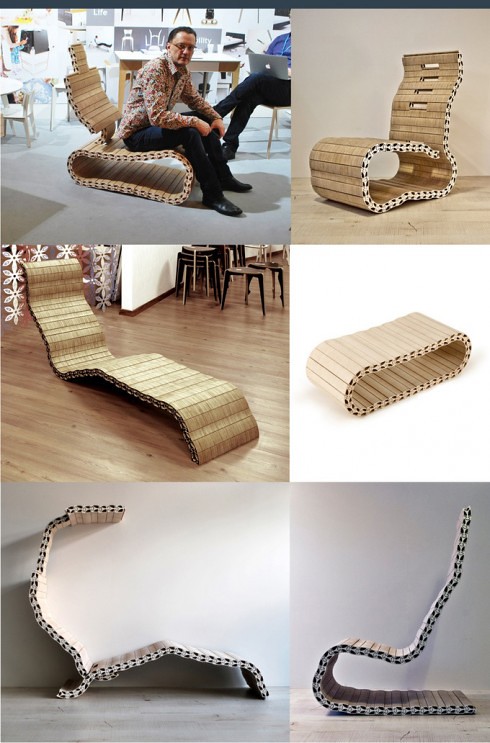This advertisement features a set of six color photographs showcasing a versatile wooden chair designed to fold into various configurations. In the top-left panel, a man in his late 50s, dressed in black pants, black shoes, and a patterned button-down shirt, is seated on the chair. The chair has an oblong wooden seat with a square backrest featuring open slots. The man is facing right, and a person with an Apple laptop is faintly visible in the background. The top-right panel highlights the chair's ability to extend its backrest, demonstrating its flexibility.

In the middle-left panel, the chair is fully reclined into a lounge chair position on a light wooden floor, with small brown step stools visible in the background. Adjacent to this, the middle-right panel depicts the chair folded into a compact, oval shape. The bottom-left panel shows the chair with a curved top extending over, resembling a lounge chair with a cover, silhouetted against a white backdrop. The final bottom-right panel presents the chair in yet another configuration: flat on the ground with the backrest curved upward to provide support. This series of images effectively illustrates the chair's innovative design and adaptability.